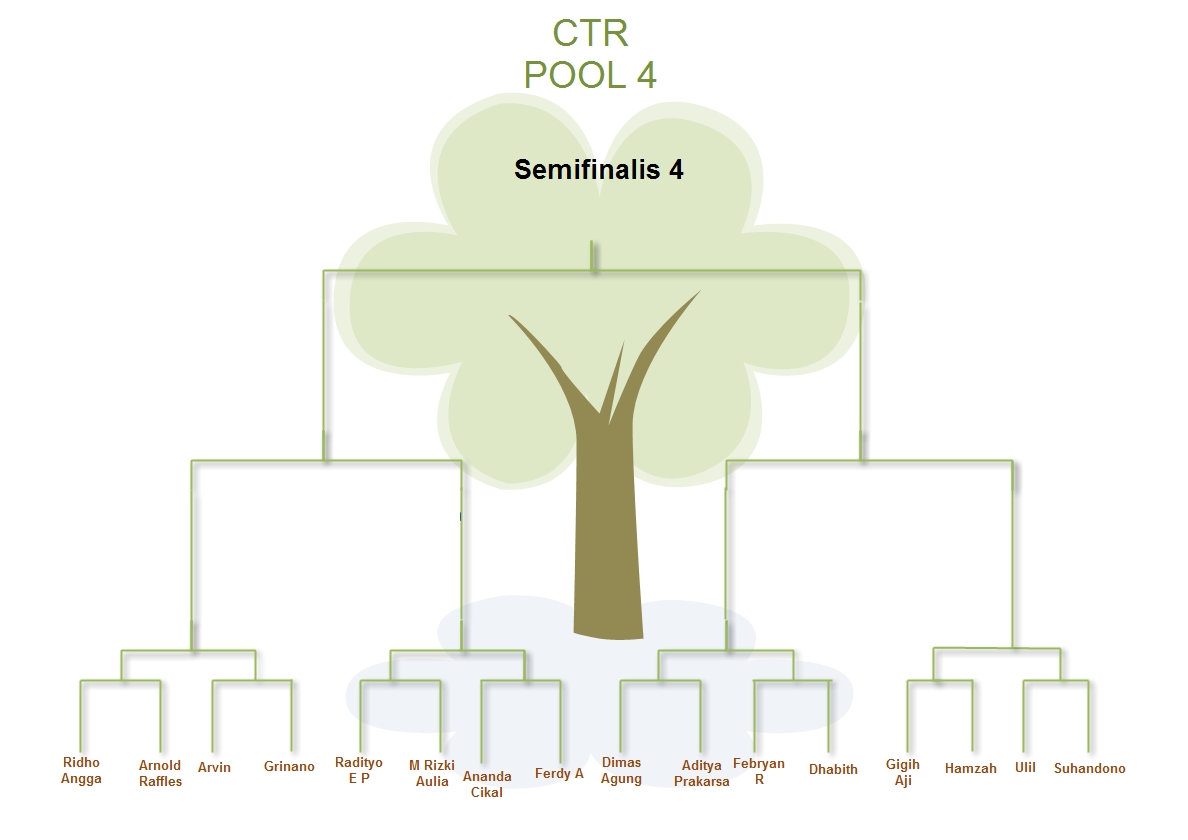This image is a digitally created poster, likely for a tournament bracket labeled "CTR Pool 4 - Semifinals". The primary visual element is a stylized tree on a white background, with a brown trunk and very light green, almost cloud-like circles representing the treetop. The tree is accented with a light blue shadow to add depth to the leaves. At the top center of the tree, "CTR Pool 4" and "Semi-finals" are displayed in green and black lettering respectively. The tree serves as a structural guide for the bracket, which starts at the bottom with multiple participants' names in orange-red font. As participants advance, the bracket narrows upward until it reaches the top, resembling the tree's structure. The entire design, including the graph with multiple legs and extensions that narrow towards the middle and top, has been digitally created using software.